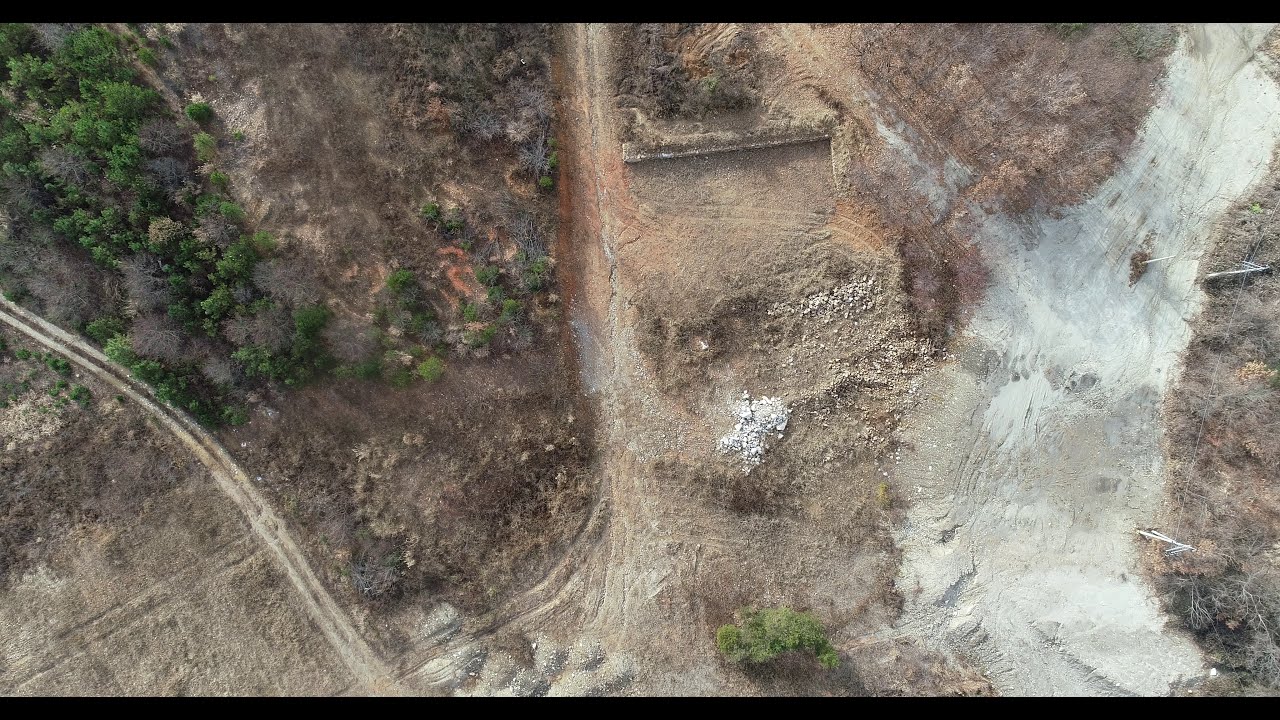This horizontal rectangular image is an aerial view, likely taken by a drone, of an urban area undergoing significant construction, set against a landscape that suggests mixed environmental conditions. The clarity of the photograph is low, making specific details hard to distinguish, but several key elements are evident. 

In the middle right section, there is a large area marked by white, curved patches, indicating a potential new road or major construction work. Adjacent to this, to the center-left, there is another construction zone, characterized by brown, barren-looking land. Surrounding these central areas, various dirt roads and tire tracks can be seen, weaving through the scene, especially prominent in the center and right sections.

On the far left of the image, a built-up urban landscape is visible, with identifiable roads and buildings. One of these roads appears to be a four-lane street running along the left side of the area, with possibly another multi-lane road wrapping around the scene.

The left edge of the image also shows pockets of green, forested areas, contrasting sharply with the brown and seemingly dead or deforested middle sections. This stark contrast suggests possible environmental degradation, such as deforestation or the aftermath of a forest fire, indicated by white and gray deposits that might be ash.

Overall, the image depicts a complex mix of urban development, construction, and contrasting environmental conditions, revealing both human impact and natural features within the same frame.